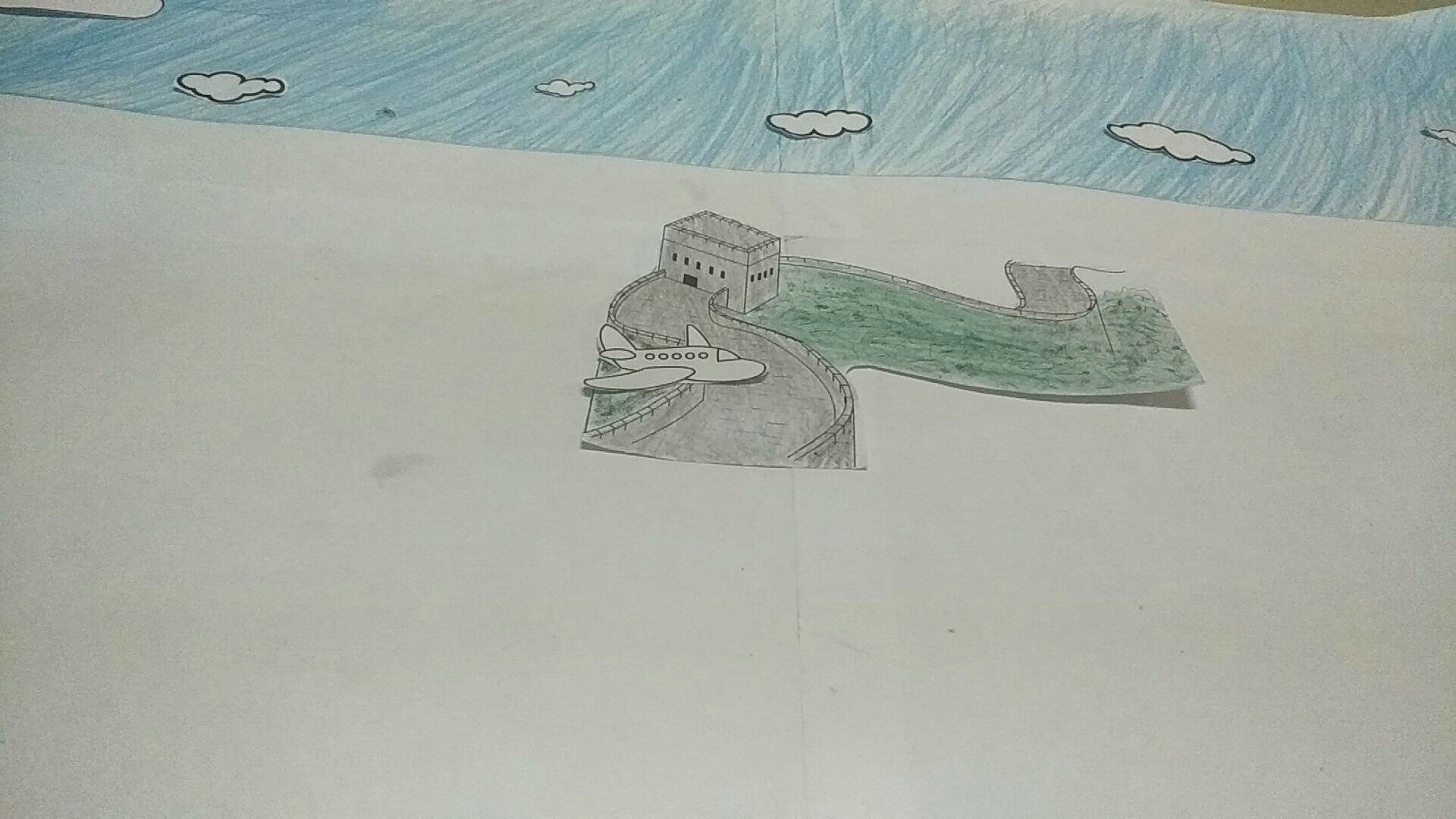This intricate drawing on a large sheet of butcher block paper exhibits a curious juxtaposition of eras and elements. At the foreground, a modern white airplane is depicted as if perched on a stone walkway that leads to a grand, medieval-style castle. The castle, rendered in shades of gray, stands robust and square, evoking a sense of historical majesty. The background is a lush green landscape, contrasting vividly with the castle’s somber tones. Above, a pristine blue sky dotted with fluffy white clouds stretches expansively, suggesting a serene ambiance. The entire scene is meticulously colored, likely with crayons or colored pencils, blending whimsy with anachronism to create a captivating visual narrative.